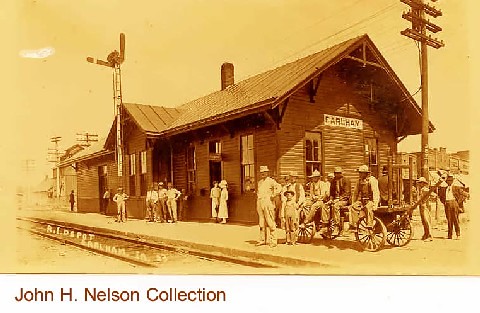This photograph, a sepia-toned image marked with "John H. Nelson Collection" at the bottom, appears to be from the 1800s, likely capturing a moment in a small Old West town. The scene centers around an old train station labeled "Earl Hay." In front of the station, at least a dozen people, including men and women, are gathered, presumably waiting for a train. To the right of the station, a wooden cart, possibly animal-drawn, holds a group of sitting men, while a few more men, one in a suit, walk toward them. Telegraph poles stretch overhead, their wires running parallel to the building. Surrounding the station, beyond its structure, a few additional buildings hint at the modest size of the town. The sky in the background is a buttery yellow, adding a timeless quality to the scene, which is punctuated by a small, flattened white cloud in the top left corner. The men in the photograph wear white hats, and the women are dressed in white, lending a uniform, almost celebratory feel to the gathering. The image vividly captures a slice of life from a bygone era, rich with community and anticipation.